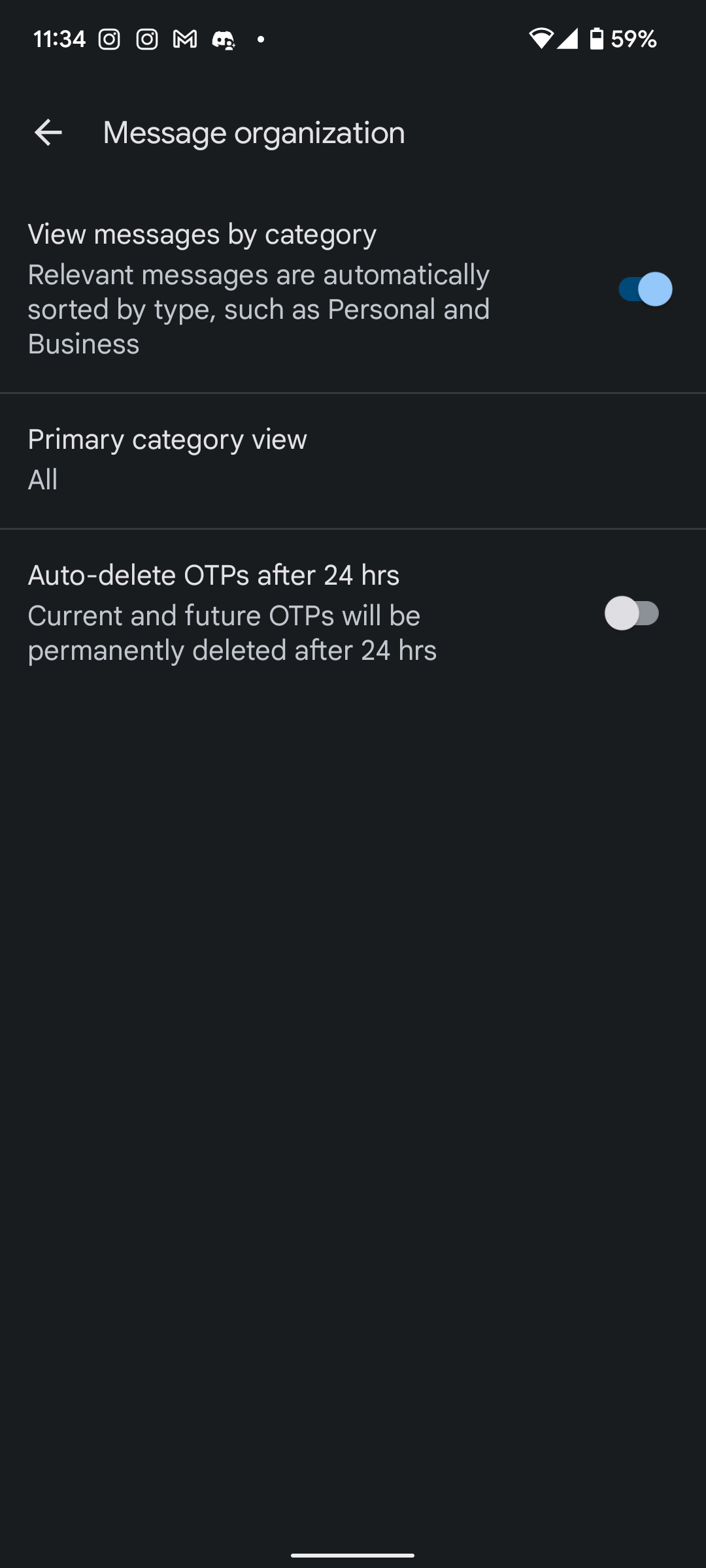This is a detailed screenshot from a cell phone displaying a settings menu. The background is black, making the white text and icons easily readable. At the very top of the screen, the status bar is visible. On the left side of the status bar, the time is shown as 11:34. Adjacent to the time are two shapes resembling Instagram logos, followed by an icon representing Google Mail (an 'M' shape), and a shape that looks like a game controller whose exact function is uncertain. Moving further to the right, there is a white dot.

On the far right-hand side of the status bar, there are icons indicating that the device is connected to Wi-Fi, showing full signal strength with four bars, and a battery icon displaying that the battery is at 59%.

Below the status bar, a category header reads "Message Organization," accompanied by a left-pointing arrow on the left side and the words "Message Organization" on the right side of this header. Directly below this header, there is a block of descriptive text stating, "View messages by category. Relevant messages are automatically sorted by type such as personal and business." Next to this description is a toggle switch that is turned on—indicated by its blue color and right position.

Further down the screen, a new section appears titled "Primary Category View," with the word "All" displayed underneath.

Another section follows, labeled "Auto delete OTPs after 24 hours." It includes the explanatory text, "Current and future OTPs will be permanently deleted after 24 hours." This section features a white toggle switch to the right, which is currently not activated.